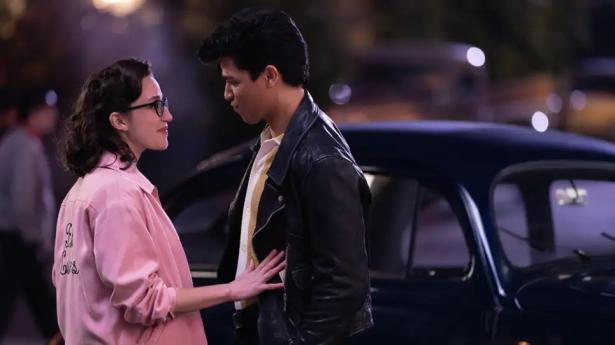The vibrant, full-color image appears to be a still from a movie, set outdoors with artificial lighting. Dominating the scene is a black 1950s-era car placed horizontally in the frame, slightly blurred to focus on the characters in the foreground. To the center left, a person in a gray jacket walks towards the right, their profile visible. In the lower left portion, a dark-haired Hispanic man, clad in a black leather jacket over a white collared shirt, stands next to a Caucasian woman. The woman, sporting black-framed glasses and a pink jacket with sleeves rolled up to her elbows, places her right hand on the man's side. Their interaction suggests they are facing each other, with the man slightly grinning and the woman smiling. The background features blurred lights and figures, hinting at a nighttime setting, with additional visible elements such as pavement through the car's windshield.